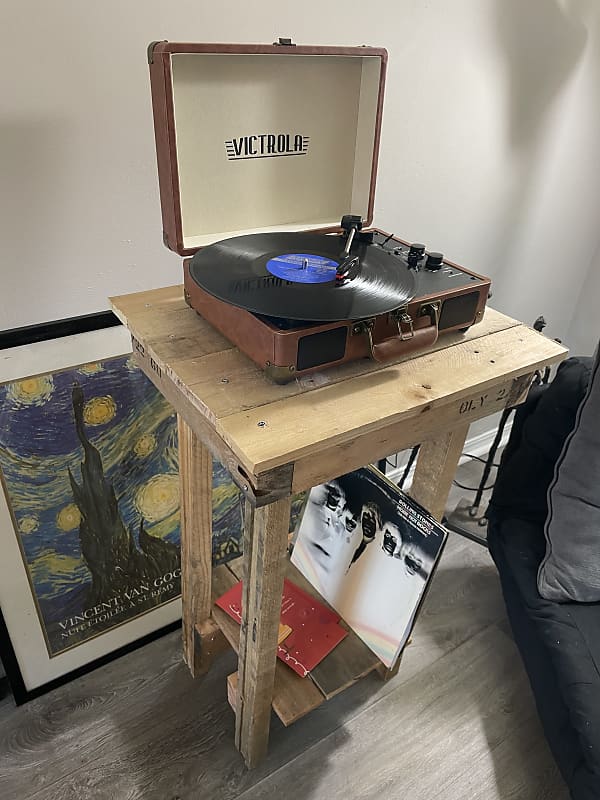The image depicts a detailed scene centered around a vintage-style record player designed as a brown leather briefcase. The Victrola record player, with its lid open displaying "VICTROLA" in black letters, is playing a black vinyl record on top of a tall wooden desk. Below this desk, several other records are neatly stacked. Part of a futon with a black cover and a gray pillow can be seen on the left side of the image. At the back, propped against a white wall, is a large painting featuring swirls, identified by an inscription as a work by Vincent Van Gogh. The image is brightly lit with natural light, providing clear visibility of the entire setup.